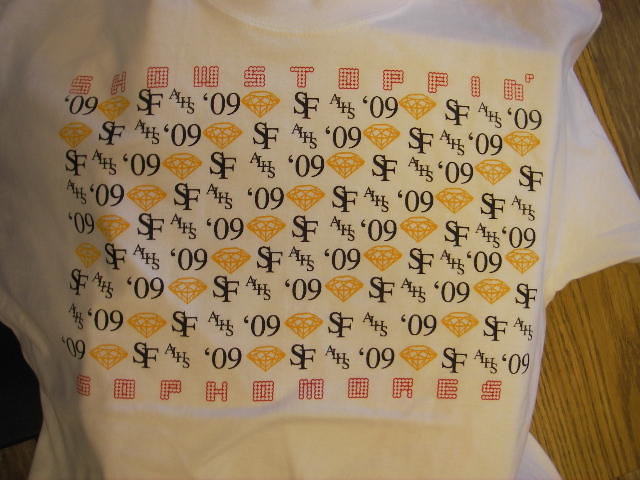This is a horizontally aligned photograph capturing a piece of fabric, likely a folded white t-shirt or tote bag, displayed on a light brown wood table. The fabric features a bold, eye-catching screen print design. At the top, in red outlined white letters, it reads "SHOW STOPPIN" and at the bottom, it reads "SOPHOMORES" in matching font. The main body of the fabric showcases a repetitive pattern comprising the letters S-F-A-H-S and the numbers 09 in black, interspersed with yellow diamonds that form diagonal lines across the fabric, adding a vibrant touch to the detailed design. The overall background of the fabric is white, enhancing the contrast and visibility of the elaborate print.